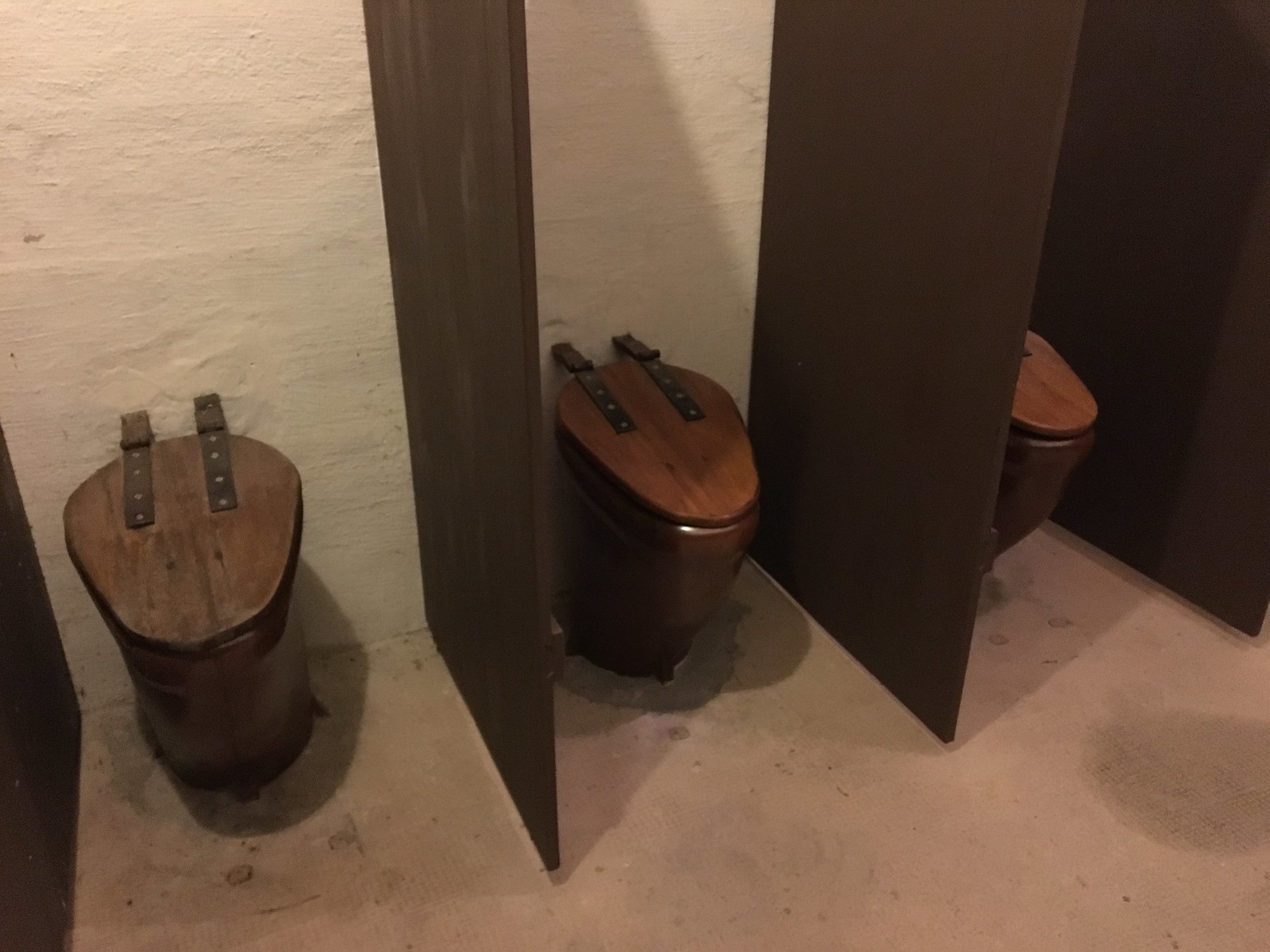This photograph depicts a well-lit restroom featuring three rustic-looking toilets arranged in semi-stalls without doors. Each stall is separated by dark brown, almost wooden, partitions. The toilets themselves appear to be fashioned from reclaimed materials, resembling old horse feeding stations turned into commodes. Each toilet has a dark wood lid, securely attached to the white wall by black metal brackets with four holes. The lids on all toilets are closed. The white wall behind the toilets is roughly finished, and the concrete floor is unfinished and gray, showing a rather stark look. There is also an apparent wet spot in front of one of the toilets and a small black stain on the floor in the bottom right corner. The overall setting gives off a rustic, somewhat industrial vibe, with elements suggesting that the toilets may not be functional or connected to a water source.